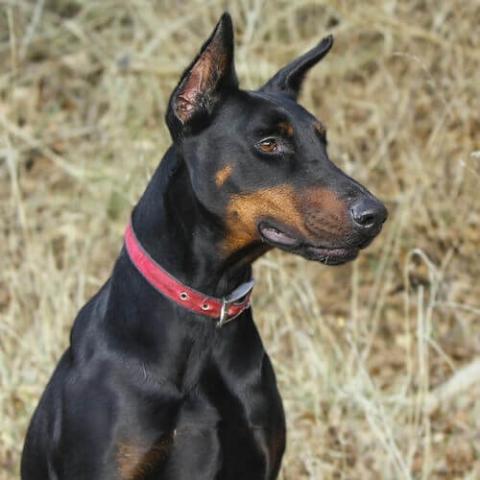This is a detailed photograph of a Doberman Pinscher, characterized by its sleek black fur with light brown patches on its muzzle and legs. The dog, which appears to have undergone the ear cropping procedure resulting in its pointed, alert ears, is wearing a weathered red collar with a silver buckle. It is positioned chest-up, with its head centrally framed but turned to the right, staring intently at something off in the distance. The dog exudes a sense of alertness and friendliness, with its slightly open mouth conveying a relaxed demeanor. The background is a blurry mix of dead grass, straw, sticks, and crunchy yellowish-tan leaves, creating a rustic and serene outdoor setting. The atmosphere behind the dog remains indistinct, leaving an air of mystery about what might be capturing its attention.